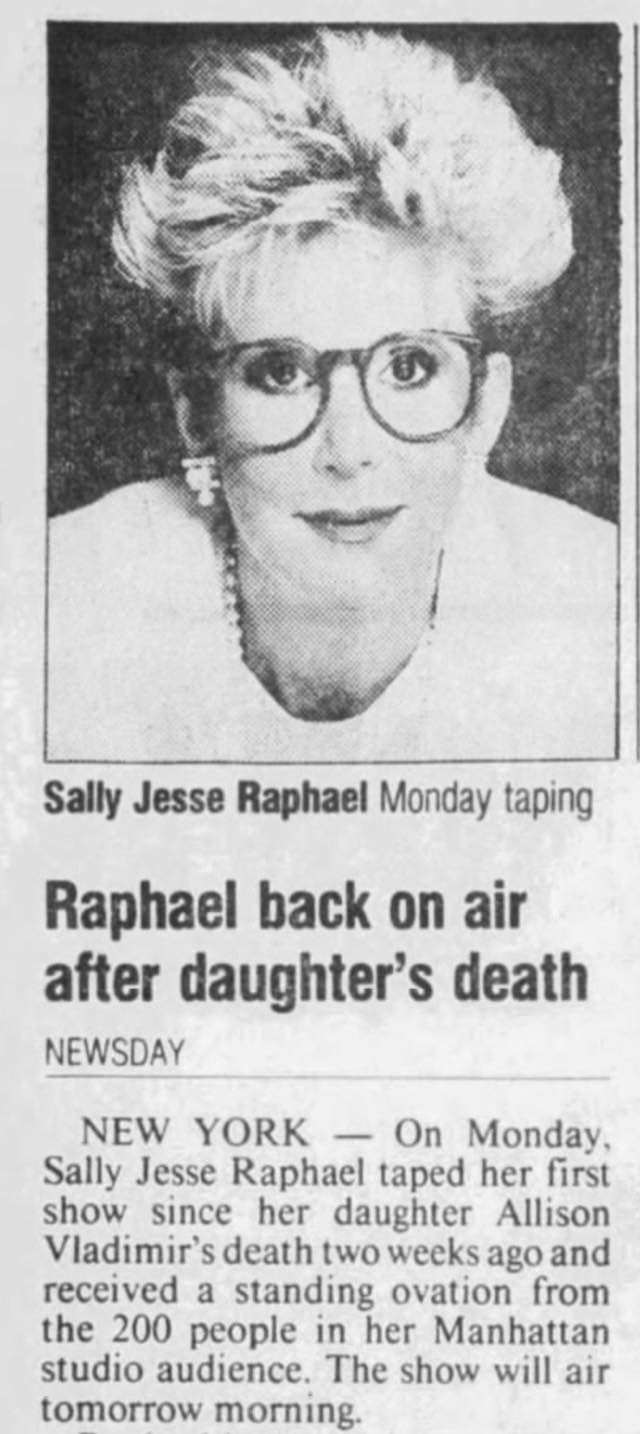The image is a black-and-white photocopy of a newspaper article featuring the talk show host Sally Jessie Raphael. Prominently displayed at the top is a black and white photo of Raphael, easily recognizable by her spiky blonde hair and signature large, round-rimmed glasses. She is dressed in an 80s style, wearing a white blouse, a pearl necklace, and earrings. The caption beneath the photo reads, "Sally Jessie Raphael, Monday taping." The headline of the article states, "Raphael back on air after daughter's death." The text explains that on Monday in New York, Sally Jessie Raphael taped her first show since the death of her daughter, Allison Vladimir, two weeks prior, and received a standing ovation from the 200 people in her Manhattan studio audience. The show is scheduled to air the following morning. The overall image, despite being a photocopy, is very clear and detailed.